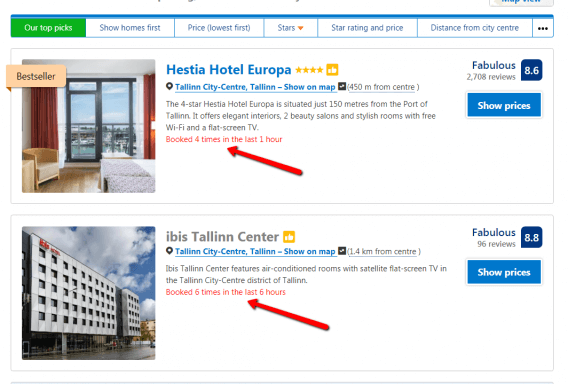"On this webpage, the top section features multiple navigation tabs, each labeled with different sorting options. The first tab on the top left is green and labeled 'Our Top Picks', while the remaining tabs are blue and read as follows: 'Show Homes First', 'Price Low to High', 'Star Ratings', 'Price', 'Distance from City Center'. 

At the bottom of the page, there are two highlighted advertisements for hotels.

The first advertisement, marked with a 'Bestseller' sticker on the left, promotes the Hestia Hotel Europa. This hotel has a four-star rating illustrated by yellow stars. It is located in Tallinn city center, specifically 150 meters from the center and just 150 meters from the port of Tallinn. The text providing this information is blue, while the description text is black. The description highlights features such as elegant interiors, two beauty salons, stylish rooms with free Wi-Fi, and a free screen TV. The advertisement notes in red text, accompanied by a red arrow, that the Hestia Hotel Europa was booked four times in the past hour. There is a blue button on the left that says 'Show Prices'. The hotel has received 2,708 reviews with an overall rating of 8.6, displayed in blue.

The second advertisement, for the Ibis Tallinn Center, specifies a location in the Tallinn city center, one kilometer from the center. The description notes that the Ibis Tallinn Center offers air-conditioned rooms equipped with satellite first screen TVs in the Tallinn city center districts of Tallinn. It has been booked six times in the last six hours, as indicated by red text and a red arrow. This entry also includes a 'Show Prices' button on the right. The Ibis Tallinn Center boasts 96 reviews with a rating of 8.8."